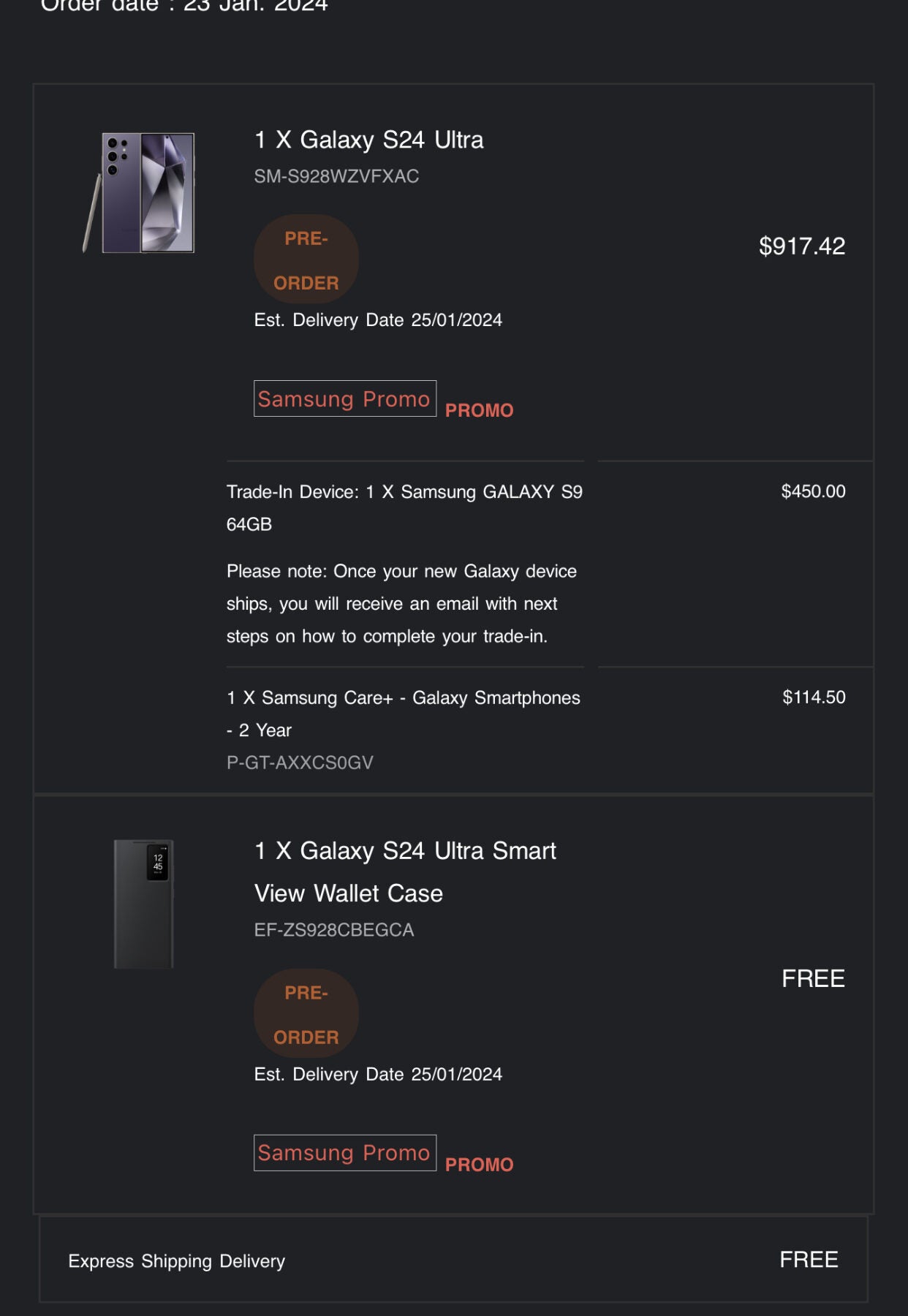A photograph taken from a cell phone screen displays a dark interface showcasing details of a Samsung Galaxy device order. The top of the image features a partially truncated text reading "Order Date: 23 Jan 2024." Below, faint gray lines outline rectangles that organize the content on the page.

The first listed item is a "1X Galaxy S24 Ultra," identified by an accompanying SM number. A circular badge labeled "Preorder" in orange text and set against an orangish background appears adjacent to this listing. To the left, a black, upright image of the Galaxy S24 Ultra is visible. The estimated delivery date for the device is noted as "25 Jan 2024."

Further details reveal that the Galaxy S24 Ultra is priced at $917.42, with an option to trade in an existing device for a credit of $450. A note informs that once the new Galaxy device ships, an email with instructions for completing the trade-in will be sent. Various clickable areas are scattered throughout the page, with one prominently displaying "FREE" at the bottom.